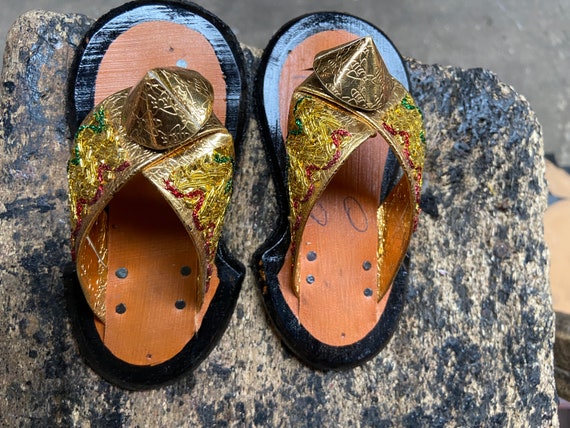In this image, two highly decorative handmade sandals with gold straps and intricate designs featuring purple, green, and gold jewels are positioned side-by-side on a heavily weathered surface. The surface, which appears almost like burnt, porous wood or degraded stone with traces of faded black paint, serves as the backdrop. The sandals have wooden-looking insoles edged in black, and each sandal is adorned with a conical gold ornament resembling small party hats at the top of the gold straps. Four nails are visible near the heel of each sandal, securing the straps to the base. The weathered background adds a rugged contrast to the ornate design of the sandals.